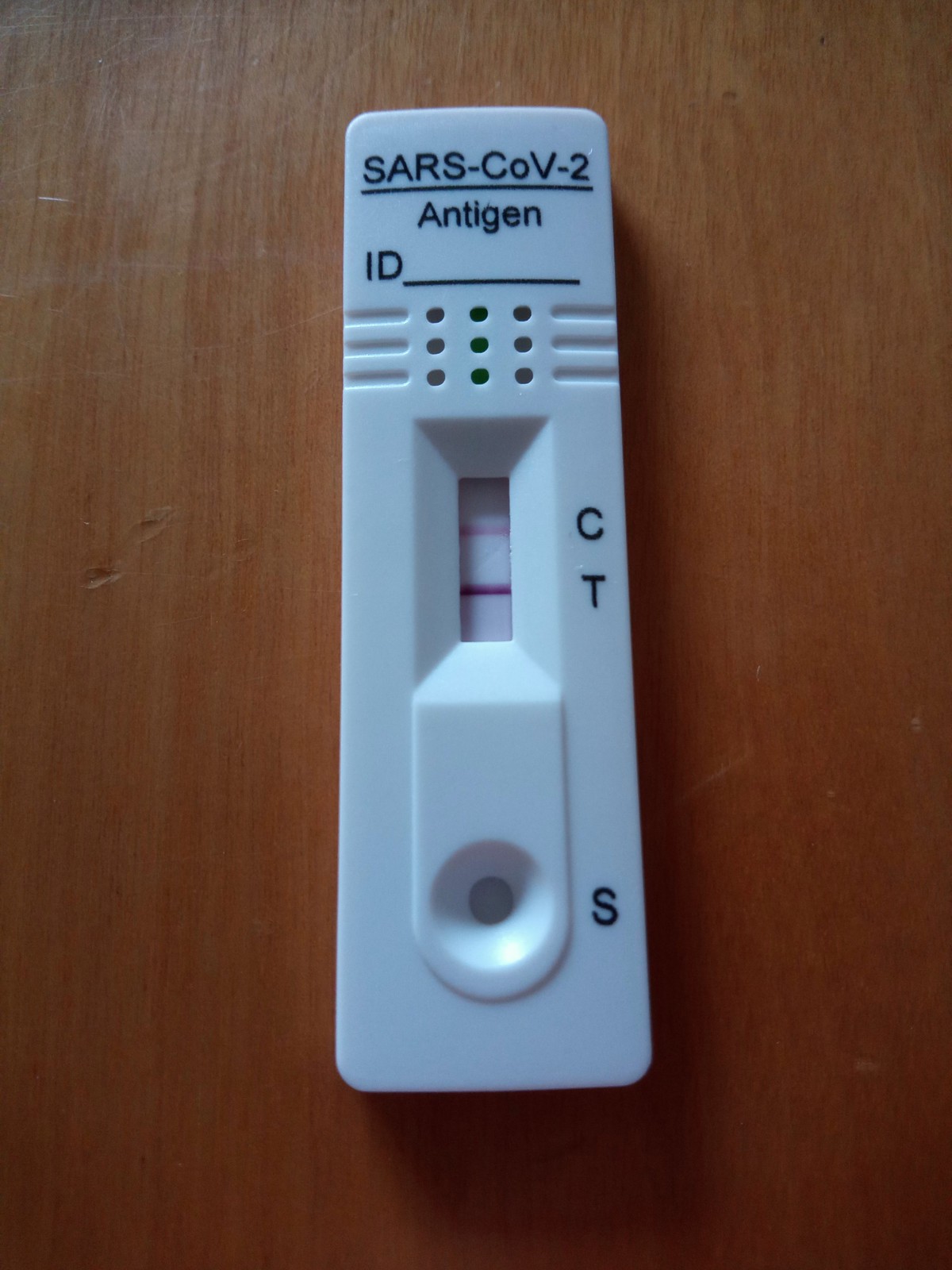This close-up photograph captures a COVID-19 rapid test laid on a light tan wooden table. The test device, a white plastic rectangular strip, dominates the image, which is oriented vertically. At the top of the device, text in white font reads "SARS-COV-2" followed by "Antigen" and "ID." Beneath these headings, a blank line is provided for writing an identification detail.

Central to the image is the test display area. The test features two distinct red lines, one aligned with the letter "C" and another with the letter "T," indicating a positive result for COVID-19. These markers are arranged vertically along the right-hand side of the test. Additionally, at the bottom of the device, a small circular inlet marked with an "S" (likely indicating the sample spot) is visible, where the test sample is deposited.

The photograph focuses solely on the rapid test device, emphasizing its details against the understated backdrop of the wooden table.